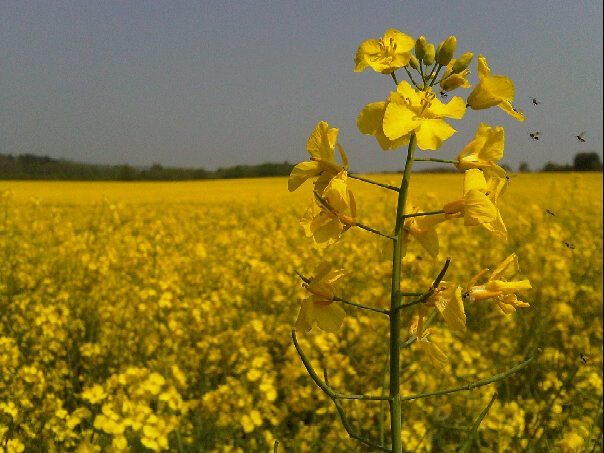This vivid photograph captures a close-up of a blossoming buttercup, its delicate, golden-yellow petals drawing attention against a vibrant green stem. The tall plant showcases a mix of open blooms and green buds that have yet to flower. Surrounding the buttercup are small, black insects with clear wings, likely in search of nectar or engaged in pollination. The right side of the image features five of these tiny insects, accentuating the scene's dynamic nature. The background fades into a soft focus, revealing a sprawling field of wild buttercups that stretch into the distance. This expansive yellow field transitions into a forested area, with lush green trees forming a picturesque horizon beneath a grey sky. The overall scene exudes a sense of natural beauty and tranquility, highlighting the intricate relationships within this vibrant ecosystem.